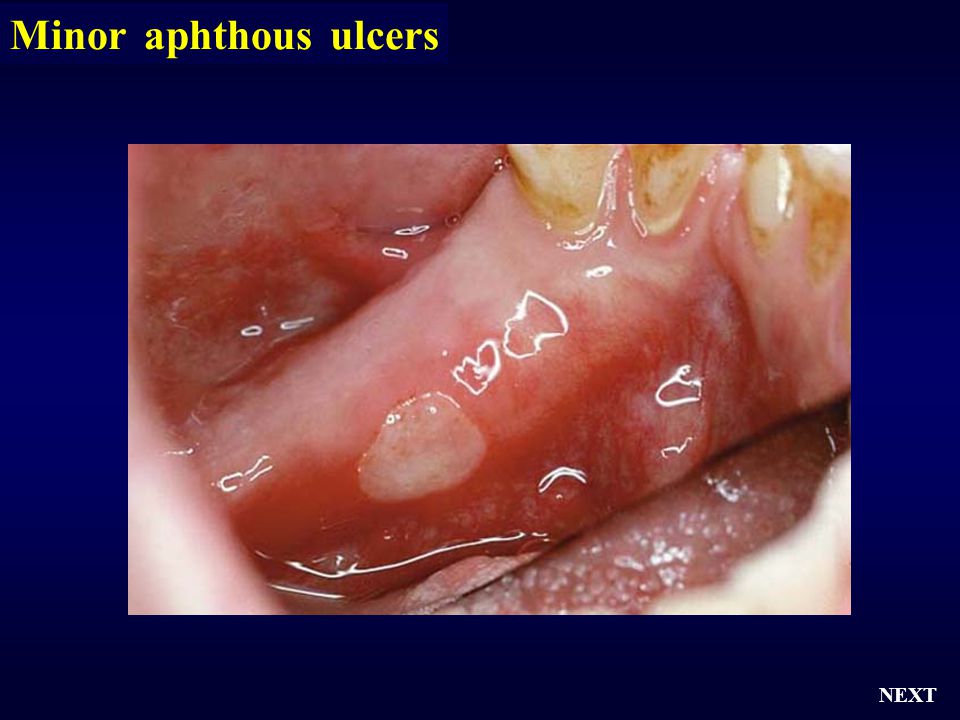The horizontally aligned rectangular image features a dark blue background, which transitions to a slightly brighter blue on the sides. In the upper left-hand corner, bold yellow text reads "Minor Aphthous Ulcers," while in the lower right-hand corner, white all-caps text states "NEXT." The central focus of the image is a close-up photograph of the inside of someone's mouth. The majority of the mouth depicted is the lower portion, showcasing part of the gum line and teeth. The gum line is wet and pink, highlighted by a prominent white patch indicative of a minor aphthous ulcer. Additionally, the person’s teeth, located in the upper right corner of the image, show noticeable brown and yellow stains, suggesting poor hygiene. The image is bordered by a thick dark blue frame approximately six inches wide and four inches tall, with the photograph in the center measuring about four inches wide by three inches tall. Part of the tongue is visible in the lower left-hand corner of the photo as it makes way for the detailed view of the ulcer.